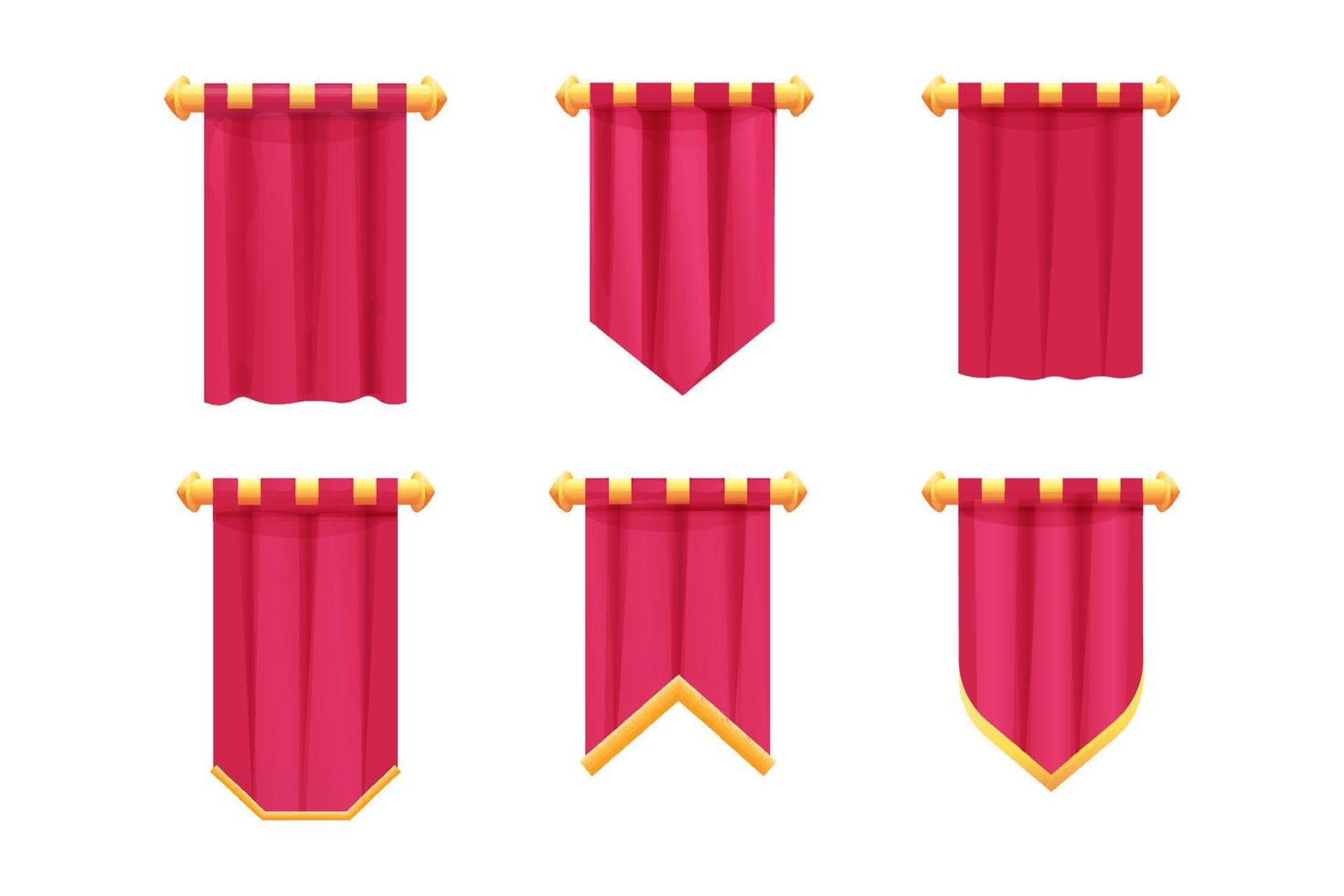The image depicts an illustration of six red banners hanging from gold-colored round rods. Arranged in two rows of three, each banner showcases a distinct bottom edge. On the top row, the left banner appears as a typical red curtain with a straight, pleated bottom. The middle banner sports a narrower tie-like shape with a pointed end. The right banner mimics the first but is shorter in length with simpler pleats. The bottom row begins with a banner on the left that features a tri-sided bottom trim in gold. The middle banner has an inverted V-shaped or reverse triangular bottom edge with yellow stitching. Finally, the banner on the bottom right displays a U-shaped bottom edge, rounded at the edges and also trimmed with gold details. Together, these banners highlight a range of historical or ancient-style designs, each unified by their red color and decorative gold rods.